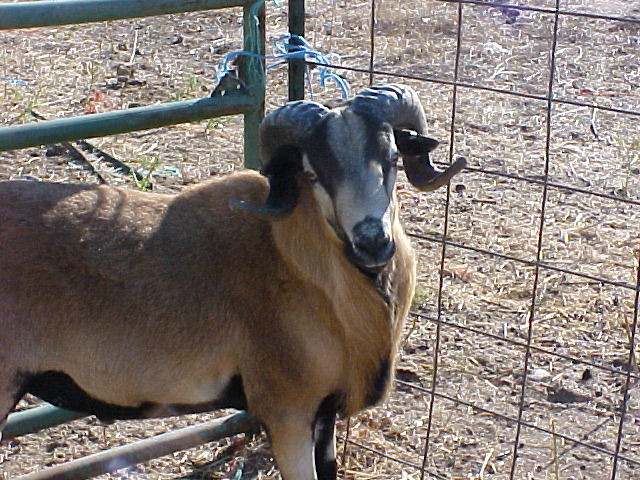This photograph, taken on a sunny day, features a ram inside a metal-fenced pen with brown, dead grass on the ground. The ram has a distinctive appearance, with a gray and black head and a body covered in short brown hair, complemented by a black underbelly. Its tall, long legs and elongated snout add to its impressive stature. The ram's most striking feature is its two large horns, which curve outward from its head, looping back towards the front. The animal gazes directly at the camera, standing near a blue rope-tied gate within the enclosure made of metal pipes and poles.